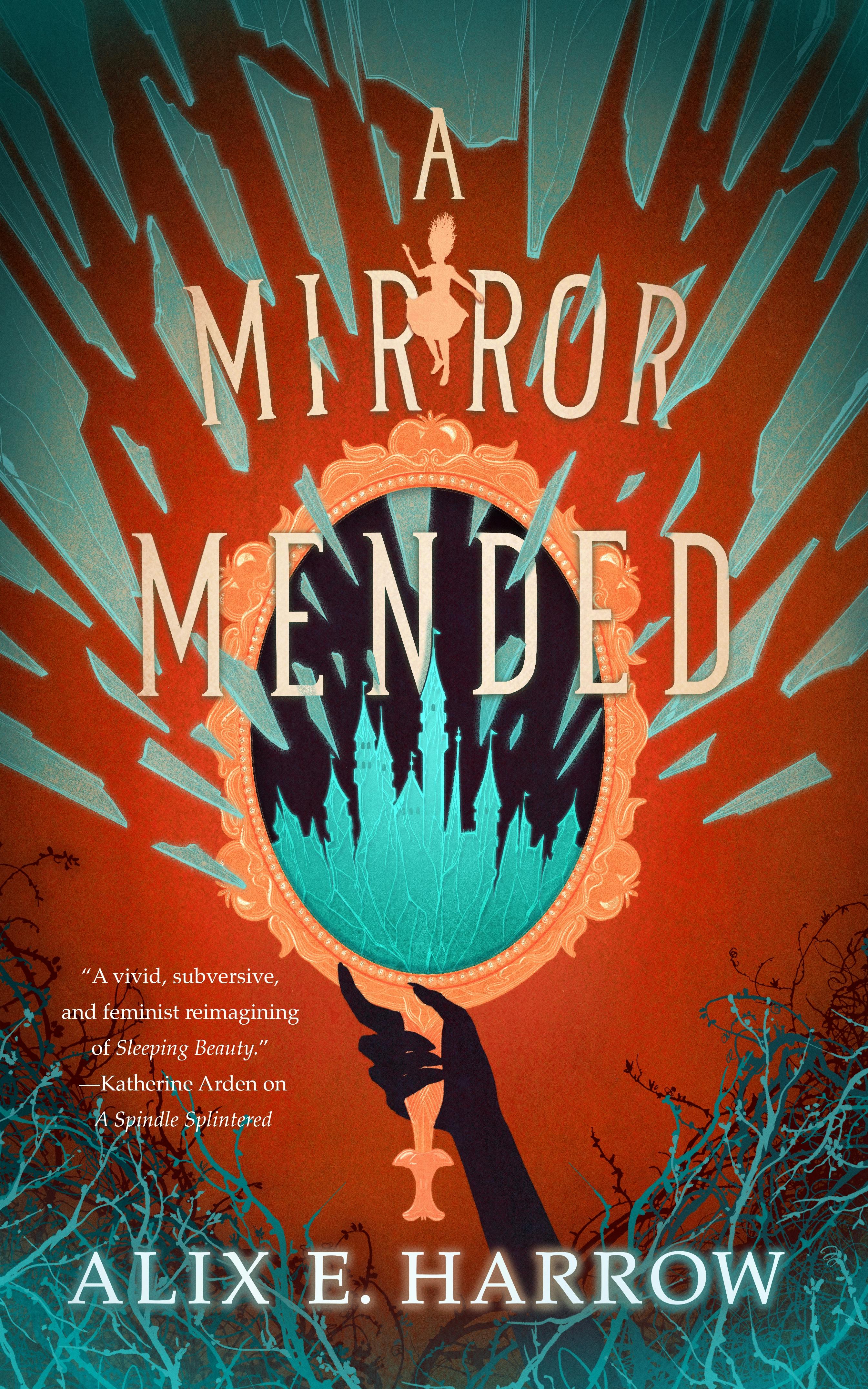The cover of the book "A Mirror Mended" by Alix E. Harrow is set against an orange background, featuring a striking black silhouetted hand at the bottom, holding up an intricate, antique-style handheld mirror with a golden frame and handle. The mirror's glass is shattered and its fragments, vivid blue in color, scatter upwards towards the top of the cover. Remarkably, the remaining shards in the center of the mirror form the silhouette of a large, castle-like structure with tall, pointed towers reminiscent of a Disney castle. Above the mirror is an outline of a woman, while a golden fairy in a dress appears between the "R"s of the word "Mirror" in the title. The book's title, "A Mirror Mended," is boldly displayed in capital white letters at the top. Towards the bottom, a quote by Katherine Arden praises it as "a vivid, subversive, and feminist reimagining of Sleeping Beauty," from "On a Spindle Splintered." This text is flanked by tree branches and vines, adding a natural, whimsical element to the cover's design.